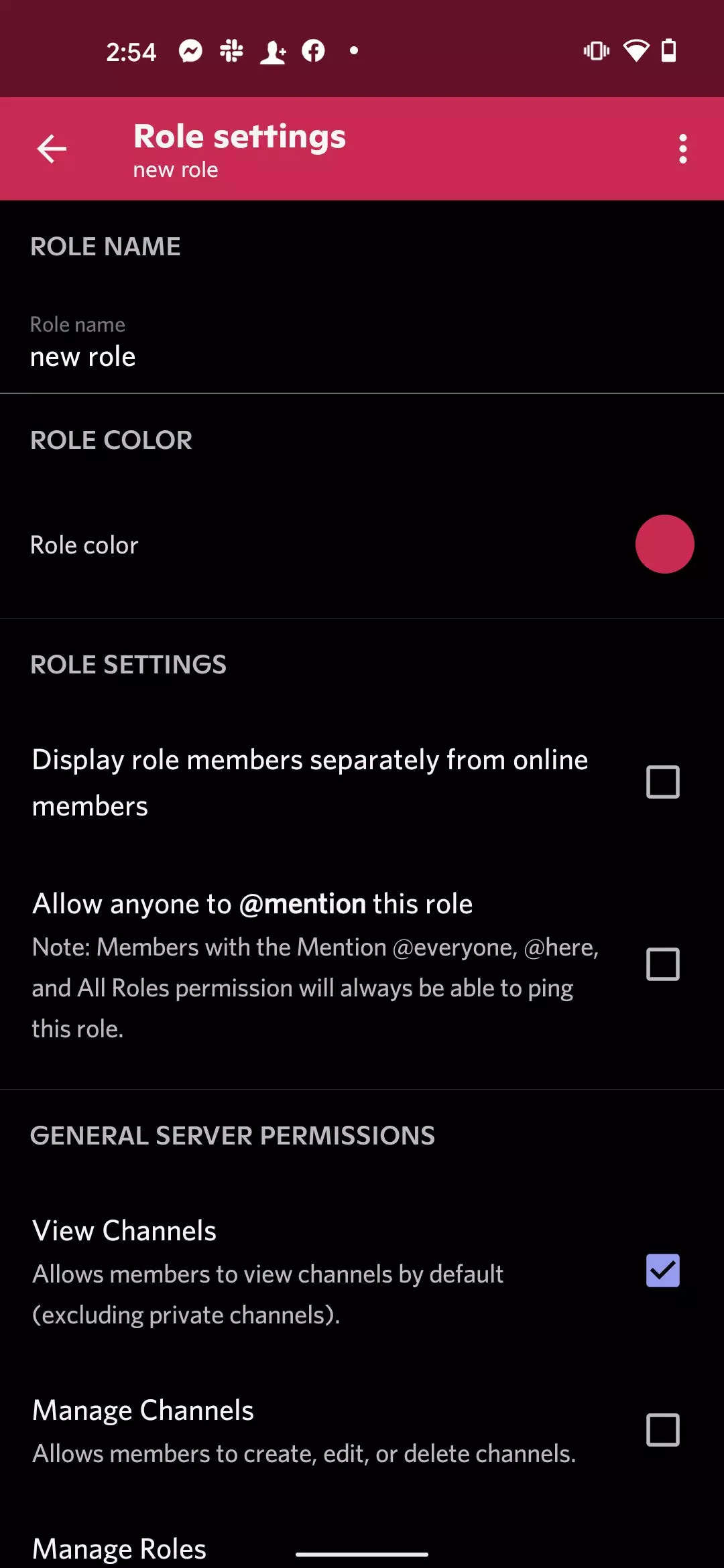The image depicts the "Role Settings" page of a mobile app in dark mode, likely designed for professional or collaborative communication, such as Discord or Slack. The interface includes a back button at the top for navigation. Below are various fields, checkboxes, and toggle switches related to the settings of a role.

- **Role Name**: By default, it is set to "New Role."
- **Role Color**: The toggle for this setting is switched on.
- **Role Settings**:
  - "Display role members separately from online members": This option is unchecked.
  - "Allow anyone to @mention this role": This option is also unchecked.

Under "General Server Permissions":
- "View Channels": This permission is checked, allowing the role to view channels.
- "Manage Channels": This permission is unchecked, preventing the role from managing channels.

While the specific term "role" might not be fully understood, it seems to signify certain permissions or designations within the app, hinting at a structured and formal communication environment for team collaboration.